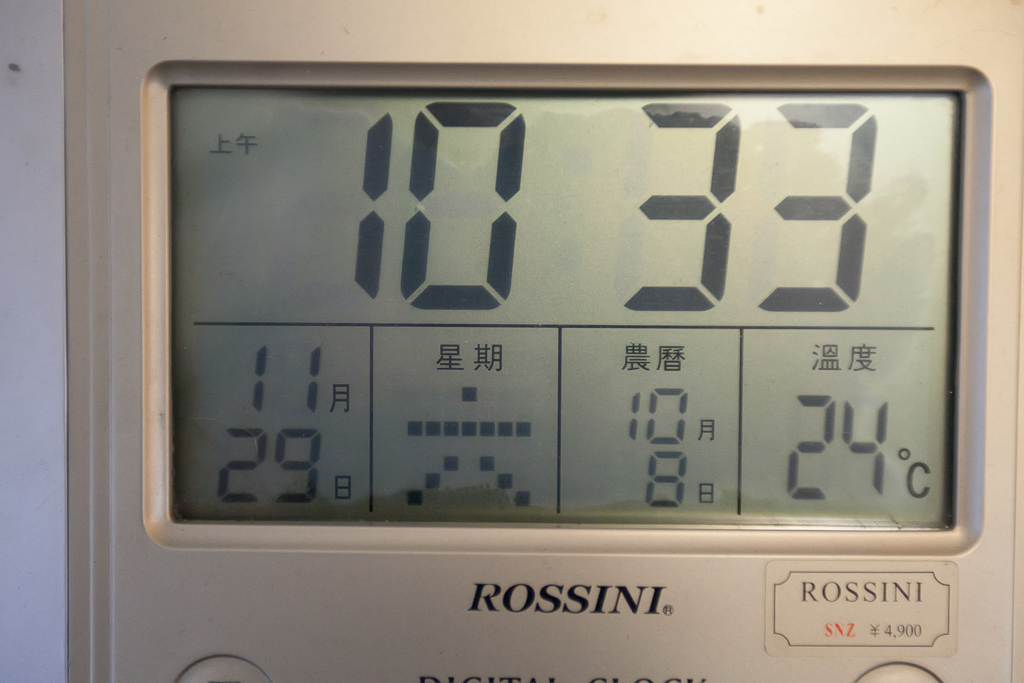This image displays a silver or gray digital clock from Japan, prominently featuring the brand name "Rossini" in black lettering below the digital readout. The main display, occupying the top half of the screen, shows the time as 10:33. In the bottom left quadrant, additional detailed readouts include the numbers 11 and 29 with some Japanese characters beside them. Adjacent to this, in the next box, appears to be a stick figure-like character, potentially another Japanese symbol. The third box contains the numbers 10 and 8, again accompanied by Japanese text. The last box on the far right displays the temperature reading of 24°C. Additionally, there is a picture resembling the Japanese currency, yen, labeled with 4900. This multifaceted digital clock provides a variety of information such as time and temperature, suggesting it functions as a control panel. The overall aesthetic is completed with some small white areas on the left side of the display.